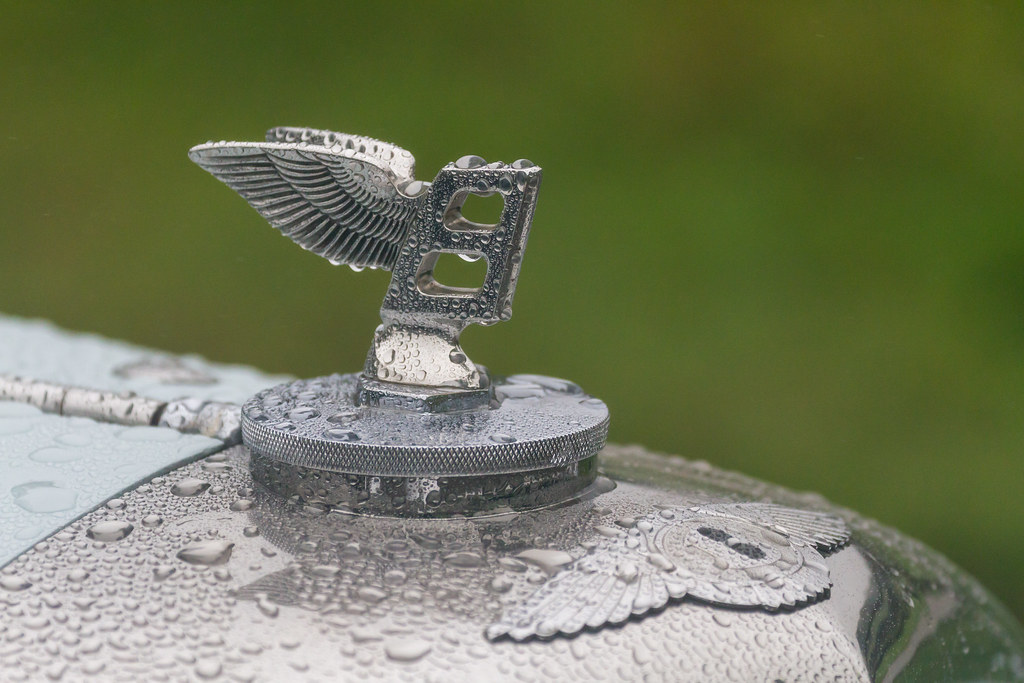This image captures a detailed close-up of what seems to be a hood ornament on a silver or gray car, which is dappled with raindrops. The centerpiece of the ornament is a silver emblem resembling an imperfect number 8 or possibly the letter B. This emblem has textured wings extending from its sides, featuring three rows of detailed feathers that add depth and interest. The emblem is mounted on a round, silver disc platform, which is edged with lines that create diagonal patterns and texture. There's a pipe-like attachment visible at the back of the round base. At the bottom of the ornament's platform sits another round logo, flanked by wings on either side, and it appears to house a bee-like figure inside. The water droplets on the car's reflective surface along with hints of green and yellow from the out-of-focus background suggest that this scene was captured on a rainy day.